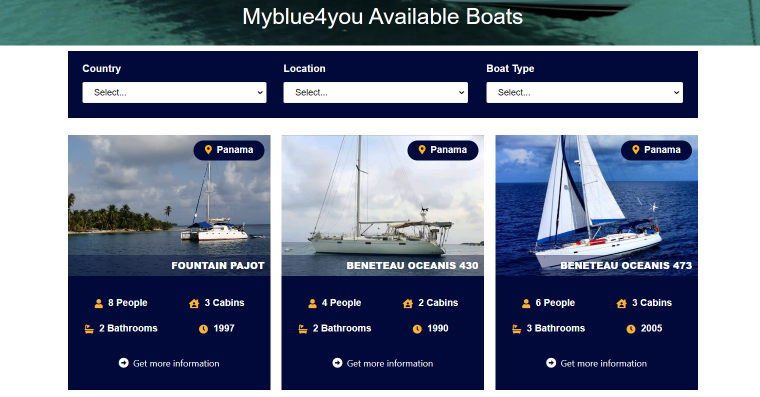The image is a screen capture of a website dedicated to renting or selling sailing boats. At the top of the image, there is a banner with a watery background, featuring the text "My Blue For You - Available Boats" in white font. Just below the banner, there is a search section that allows users to refine their search results. This section includes dropdown menus for selecting the county, location, and boat type.

Below the search section are listings for three different boats available in Panama:

1. The first listing is for a Fountain Pajot, dated 1997. It has an image of the boat anchored near an island. The boat accommodates eight people, has three cabins, and includes two bathrooms.

2. The second listing is for a Beneteau Oceanis 430, dated 1990. The accompanying image shows the boat floating in the ocean. This boat can accommodate four people, features two cabins, and has two bathrooms.

3. The third listing is for a Beneteau Oceanis 473, dated 2005. The image shows the sailing ship in motion on the ocean. This boat is suitable for six people, contains three cabins, and has three bathrooms.

Each listing provides a detailed breakdown of the boat's specifications and amenities, offering potential renters or buyers ample information to make an informed decision.